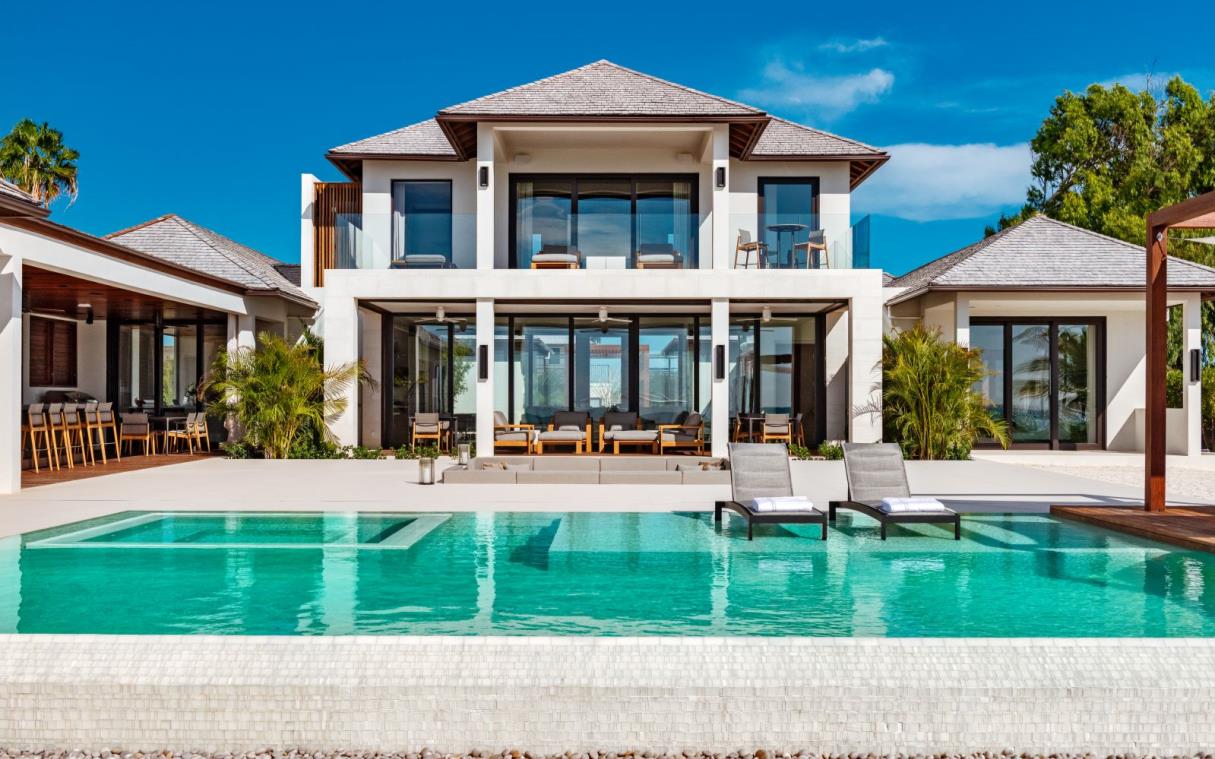The image showcases a luxurious villa featuring a stunning backyard pool that epitomizes relaxation and modern design. The sleek, rectangular pool immediately draws the eye with its shimmering blue water, flanked by strategically placed pool chairs that rest on a shallow ledge, allowing occupants to lounge comfortably without being fully submerged. The deeper section of the pool extends further into the background, offering ample space for swimming.

The villa itself is an architectural marvel, characterized by its clean, right-angled design and modernist appeal. The structure is predominantly white with light brown roofing, enhancing its neutral, cohesive aesthetic. The two-story building boasts expansive glass doors and windows, creating an open, airy feel that seamlessly blends indoor and outdoor spaces.

Both levels of the villa feature patios furnished with stylish outdoor seating, ideal for enjoying the picturesque surroundings. On the upper-level patio, a balcony with large windows offers a panoramic view of the area, while the ground-level patio invites guests to relax closer to the pool.

To the side of the main building, smaller white rental units with matching brownish roofs are visible, aligned neatly in a row. Each unit continues the theme of modern elegance. Vegetation, including the top of a palm tree, adds a touch of greenery to the otherwise minimalist landscape, underscoring the serene and well-manicured environment.

Overall, the villa presents a harmonious blend of luxury, comfort, and sophistication, making it an idyllic retreat.